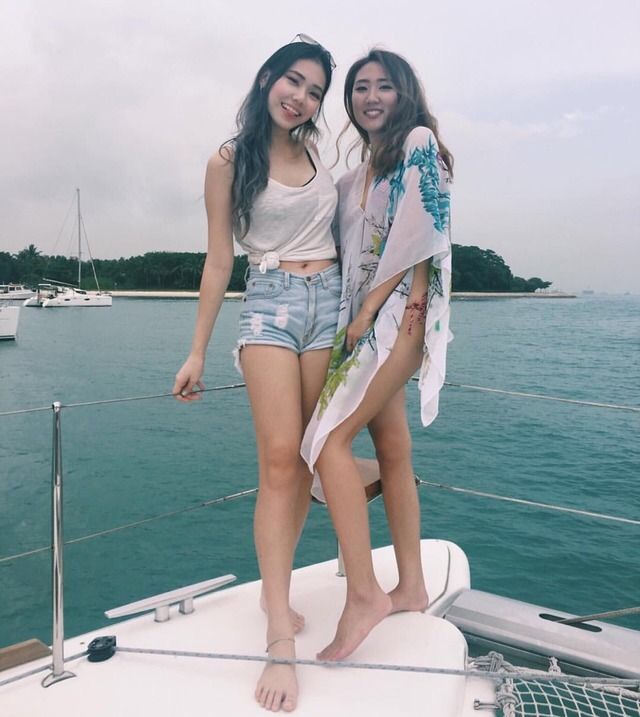In this photograph taken on an overcast day, two women are standing and posing on the bow of a white catamaran, with silver posts and cables serving as safety rails. The woman on the left, who has long black hair with sunglasses perched on her head, is dressed in a white tank top tied in the front, revealing a swimsuit top underneath, and distressed blue jean shorts. She is smiling and sticking out her tongue, holding onto one of the posts. An anklet adorns her ankle. The woman on the right, with dark hair reaching just below her shoulders, is also smiling. She wears a white swim cover-up adorned with blue and green patterns over a bathing suit, and her left leg is prominently visible. Surrounding them, the turquoise water of the ocean reflects the overcast sky. In the distant background, to the left, another catamaran is visible. Further back, a land mass with lush green trees stretches almost the entire width of the image. The sky is filled with gray clouds, indicating it is daytime.